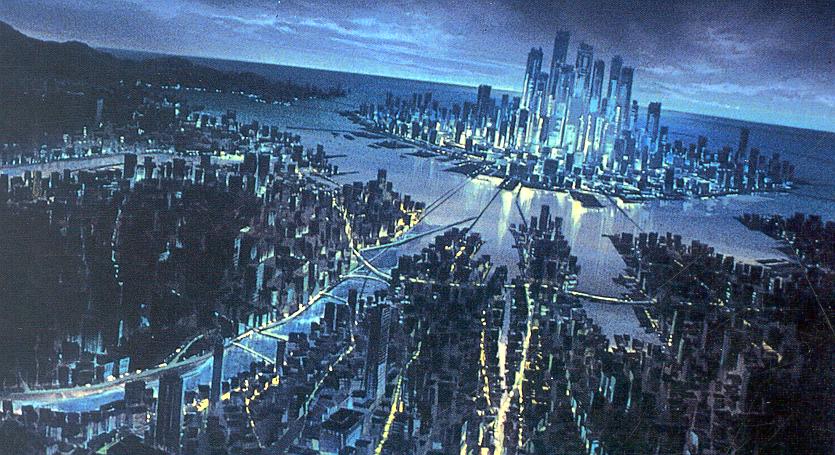A computer-generated nighttime scene depicts a sprawling metropolis, similar to a futuristic New York, centered on an island connected by bridges and roadways. The city is illuminated with cobalt blue lights, giving it a vivid yet ominous appearance under a sky filled with dark purplish-black clouds. Skyscrapers dominate the island's skyline, radiating outwards into denser areas with more buildings and stretching suburbs. Roads crisscross the landscape, leading from the wooded left-hand side towards the vibrant heart of the city. The artistic rendering, characterized by its gradient color scheme, meticulously illustrates the contrast between the bright city lights and the surrounding dark night.